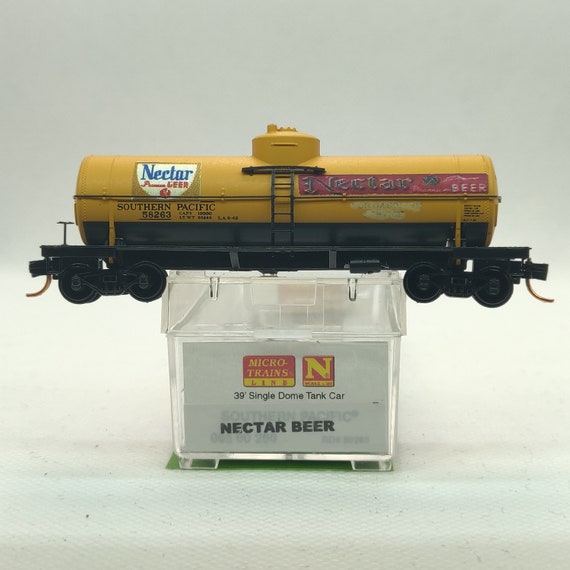The image features a detailed, small model tank car from a toy train set. The tank car is primarily a dark yellow color with a black base, resting on a black trailer equipped with two sets of black wheels at each end. The left side of the tank car displays the words "Nectar Beer" with "Nectar" in blue and "Beer" in red, alongside the labeling "Southern Pacific 58263." The right side features a red banner with the words "Nectar Beer" prominently displayed. The car includes a small ladder in the middle. The model is placed on a clear square plastic stand which bears the inscription "Micro Trains Line, 39-foot single dome tank car, Southern Pacific, Nectar Beer." The background of the image is a white or off-white cloth.